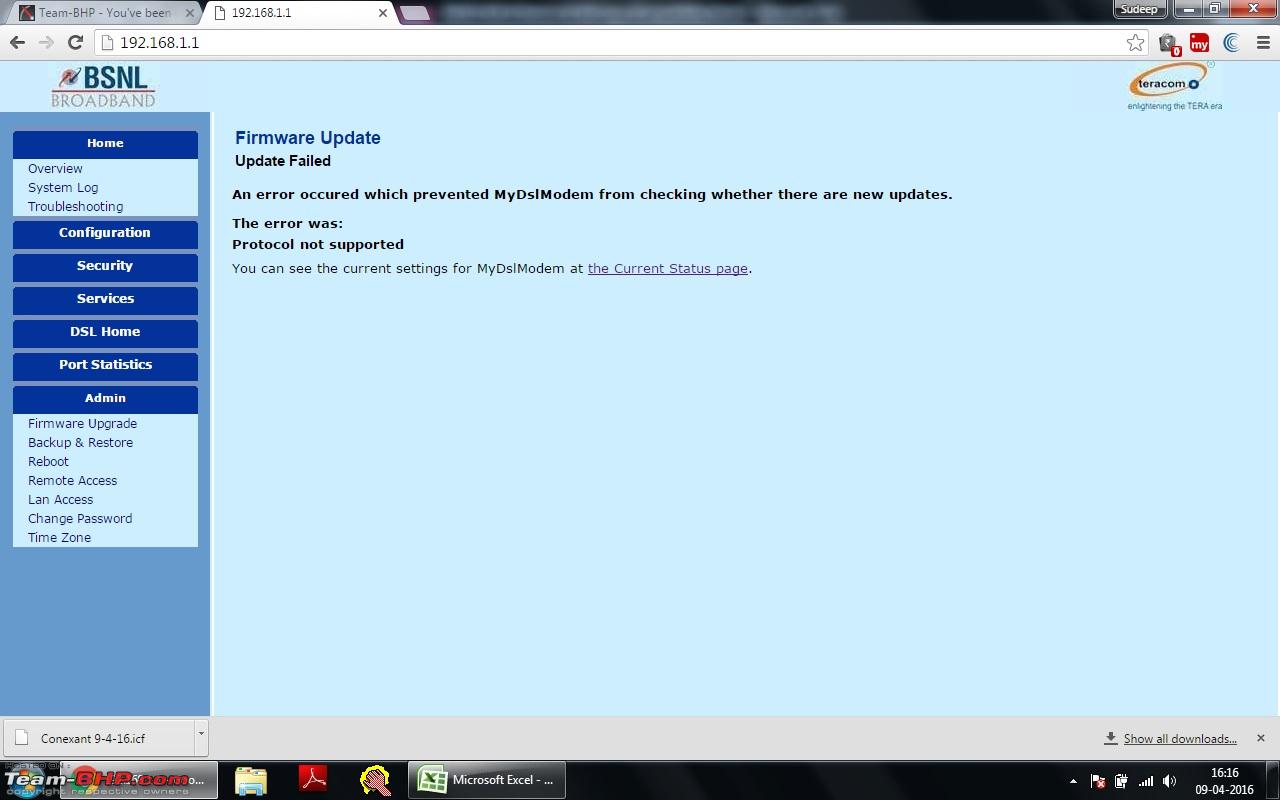This image portrays a webpage displaying the BSNL Broadband interface. In the upper left corner, the website proudly displays "BSNL Broadband." The browser's address bar reads "192.168.1.1," indicating it is accessing a local network page. Within the browser, there is a partial and unclear phrase, "TMBHP You've Been." In the top-right corner of the webpage, there is a prominent red 'X' button.

Located towards the center-right, the name "Sudeep" appears alongside a "Teracom" logo encircled in brown. The page is sprinkled with various images in red and blue.

Beneath the company name, several navigation options are listed: "Home," "Overview," "System Log," and "Troubleshooting," all housed within a light blue box bordered by a darker blue one. The layout continues with another blue box containing additional options: "Configuration," "Security Services," "DSL Home," "Port Statistics," and "Administration." These are followed by a lighter blue section featuring "Firmware Upgrade," "Backup and Restore," "Reboot," "Remote Access," "LAN Access," "Change Password," and "Time Zone."

The main content area of the webpage is light blue and includes a message in purple that provides important information: "Firmware Update: Update Failed. An error occurred which prevented MyDSI Modem from checking whether there are new updates. The error was Protocol Not Supported. You can see the current settings for MyDSI Modem at the current status page." This message includes a clickable link for "current status page."

At the bottom of the screen are several advertisements and icons. Additionally, there is an option to "Show all downloads."

Overall, the image meticulously captures the intricate and detailed layout of a technical and navigational interface for BSNL Broadband.